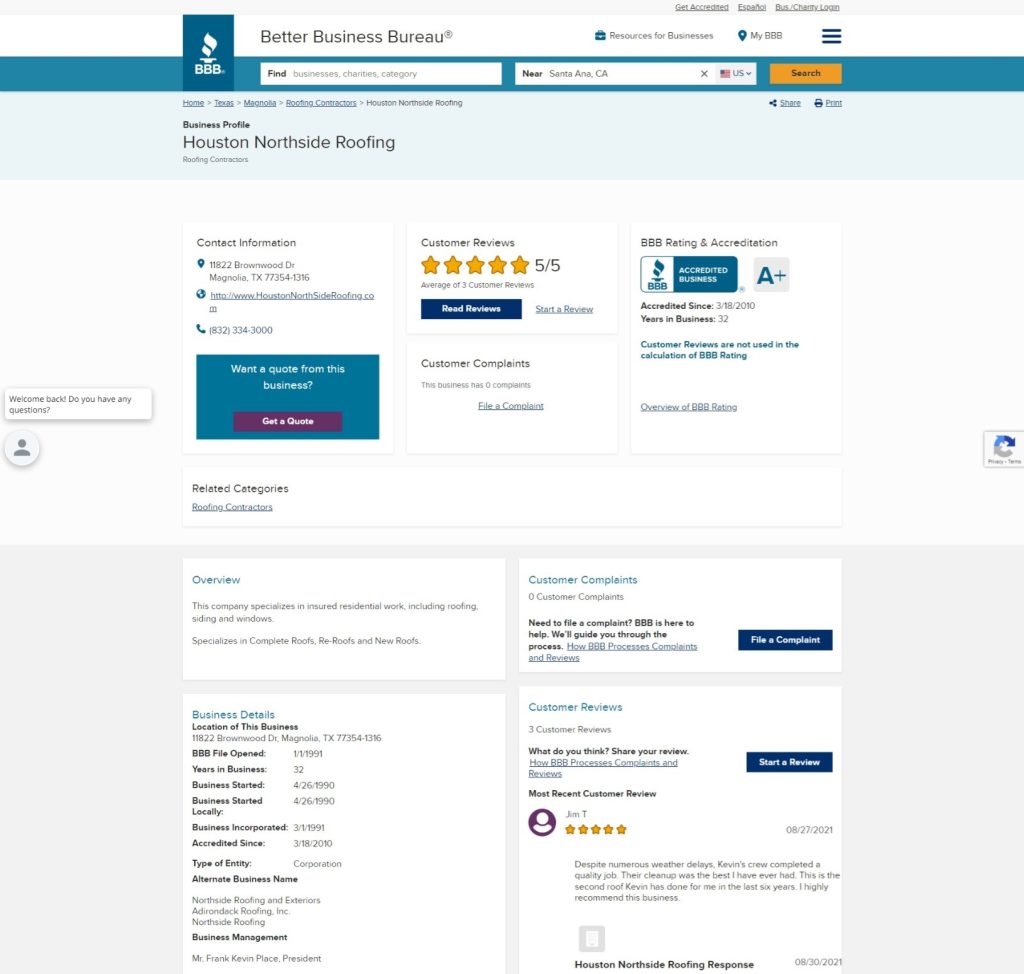This screenshot from the Better Business Bureau (BBB) website provides a detailed overview of "Houston Northside Roofing." In the upper left corner, the BBB's blue box logo is prominently displayed, while the upper right corner features light gray text options for "Get Accredited," "Español," "Bus," "Charity," and "Login." Two search bars are visible: the first allows users to find businesses, charities, and categories, and the second specifies search locations with a suggestion of "Santa Ana, California."

The main business profile focuses on "Houston Northside Roofing," categorized under Roofing Contractors. The company boasts a perfect 5 out of 5 yellow star review rating based on three customer reviews and holds a BBB rating and accreditation of A+. The company specializes in insured residential work, including roofing, siding, and windows. The most recent customer review is highlighted: Jim T. awarded the company five stars, with a review dated August 27, 2021.